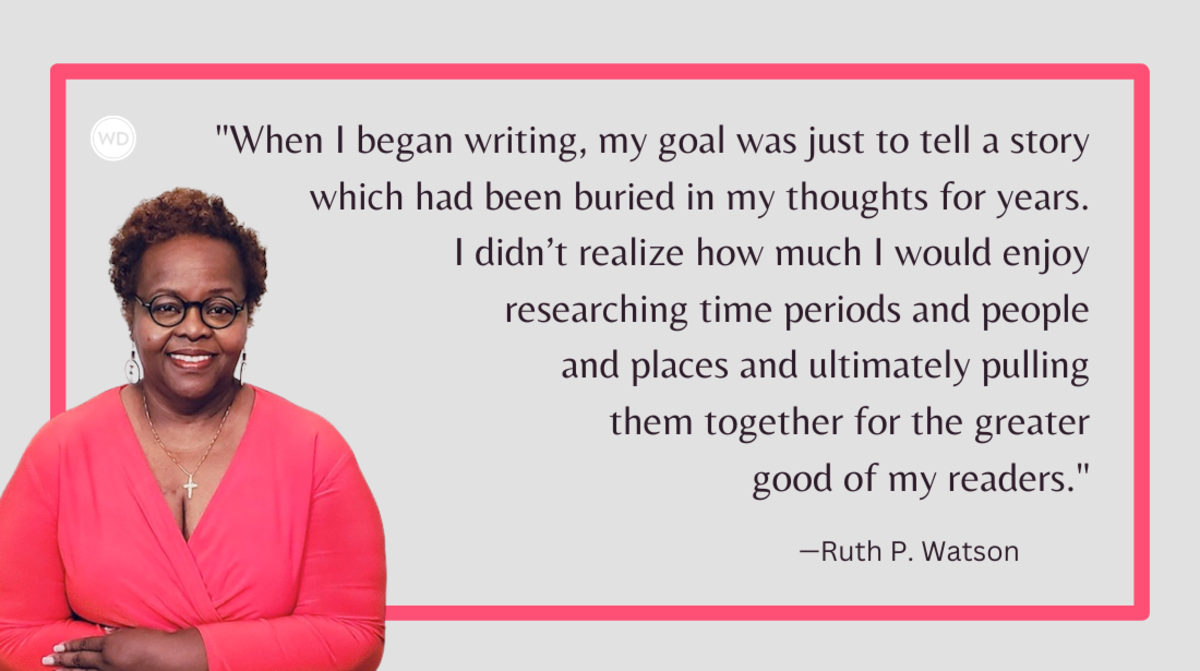The image features a light gray background with a highlighted text in a pink-colored rectangle. The text reads, "When I began writing, my goal was just to tell a story which had been buried in my thoughts for years. I didn't realize how much I would enjoy researching time periods and people and places and ultimately pulling them together for the greater good of my readers," attributed to Ruth P. Watson, with the initials "WD" in white at the upper left corner. In the bottom left of the image, there is a picture of an older, smiling Black woman with thick, curly hair that's a mix of brown and orange hues. She is wearing black glasses, red lipstick, a red long-sleeved shirt with a bit of cleavage visible, a cross necklace, and earrings. Her hands are folded in front of her. The thoughtful positioning of the woman and the text together create a sense of her connecting with her audience through her writing.